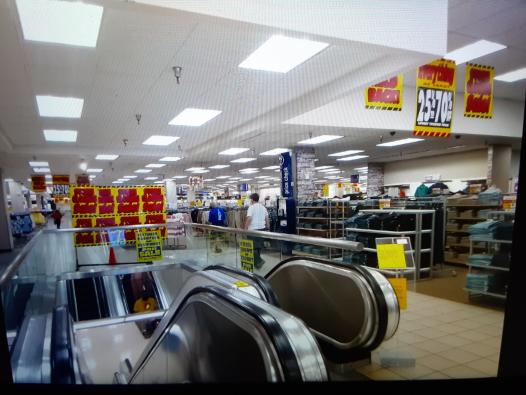The photograph captures a bustling scene inside a large, well-lit department store, likely situated within a larger mall. The store features white walls and ceilings, with bright fluorescent lighting running the length of the space. Beige tile flooring is complemented by tan brown carpets in some sections. Prominent in the foreground are the tops of two escalators—one ascending and one descending—encased by clear, transparent banisters.

Numerous signs are displayed throughout the store, both on the walls and suspended from metal staffs attached to the ceiling. These signs announce a "Back to School Sale" with discounts ranging from 25% to 70% off various items. The sales advertisements and the overall size of the store suggest a broad inventory that likely includes clothing, toys, electronics, and home furnishings, though in this image, the primary visible items are jeans and shirts. Shelves and clothing racks line the aisles, displaying an assortment of garments, while several shoppers meander through the aisles. The combination of escalators, spacious layout, and assortment of merchandise indicates that this is indeed a large, multi-faceted retail environment.